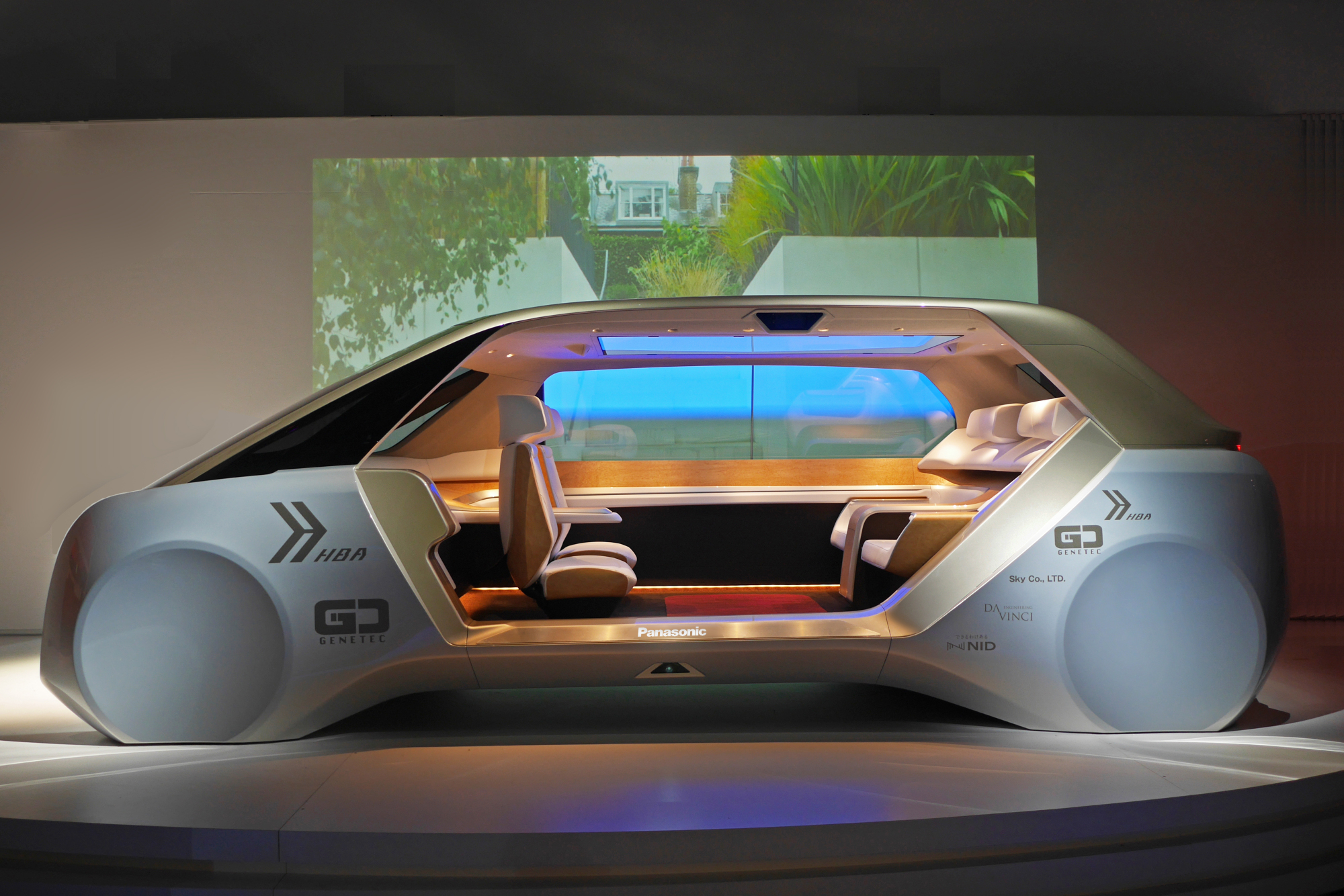This is a highly detailed photograph of a futuristic, concept car on display, likely at an auto show. The car, with a matte silver-gray finish, is displayed on a round, gray stage against a backdrop that simulates a view of buildings, green trees, and a potentially concrete fence. The scene suggests a projection that could be set up to resemble a domestic environment.

The vehicle itself boasts an unconventional and boxy design with a notably long front end reminiscent of traditional cars. However, it lacks visible car doors on the side in view, offering a clear look into its interior. Notably absent are typical black rubber wheels; instead, where the wheels would be, the car features fully covered metal hubs with a circular imprint, possibly indicating retractable wheels or an advanced hovering capability.

Inside, the car does not have a steering wheel, reinforcing the idea it may be an automated vehicle. The seating arrangement is unique, with all seats facing inward towards each other, suggesting a communal travel experience. The seats are a blend of cream and beige colors, contributing to a sophisticated look. The car is equipped with a large front and rear window, a continuous side window on the opposite side from the viewer, and a substantial sunroof spanning much of the roof.

Text on the vehicle includes several legible inscriptions: on the front side, two arrows point right towards the letters "HBA," with similar markings on the rear side. The front also features a discernible “G” and a letter resembling a backward "C," repeated on the back with additional unreadable font beneath them. Additionally, on the car’s middle base, the word "Panasonic" is prominently displayed in white font.

Further inscriptions include "Sky Company Limited," "DaVinci," "NID," and possibly "GD Genetic," adding to the mystique and high-tech allure of the vehicle. The overall impression is one of cutting-edge innovation, presenting a transport mode that defies traditional automotive design and functionality.